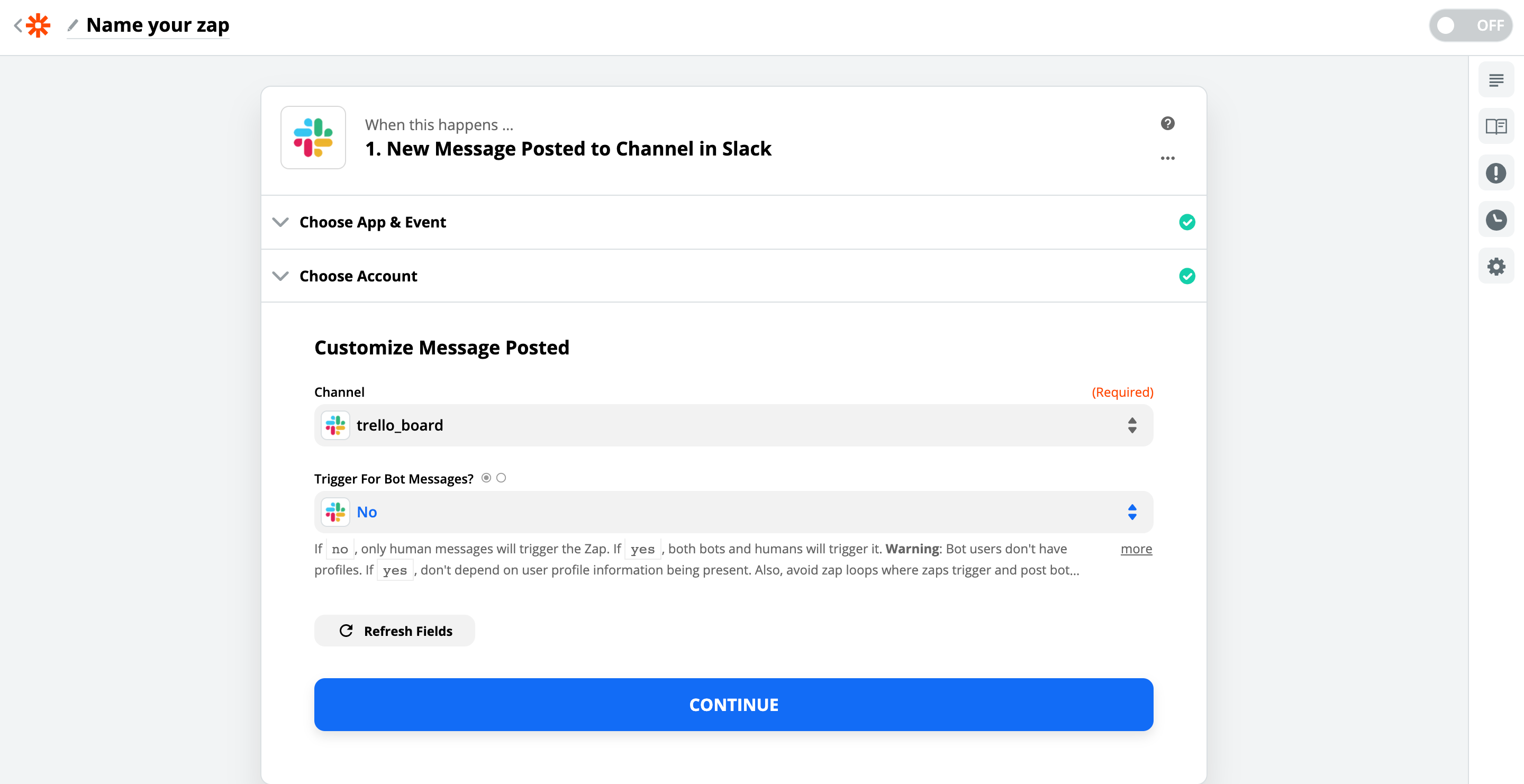Here is a cleaned-up and detailed caption for the given image description:

---

The image is a screenshot of a Slack settings screen, with a white border present at the top and right edges. 

**Top Left Corner**
- A prominent red cogwheel icon is situated at the top left, accompanied by a grey left-pointing arrow.
- Right next to the cogwheel, a small light grey pencil icon is visible, adjacent to the bold black text that reads "Name your zap."

**Top Right Corner**
- In the far right corner of the screen, there is a toggle switch with a grey background displaying the word "Off" in white letters inside the toggle.

**Right Side Icons**
- On the right side, there are five small grey boxes, each containing an icon: an exclamation point, a clock, a cogwheel, an open book, and a menu icon.

**Main Content Area**
- The central background is grey, featuring a large white box. In the top left of this box, the Slack logo is displayed.
- Below the logo, bold black text states, "When this happens, one new message posted to number one and then new message posted to channel in Slack."
- Further down, it provides setting options:

  - **Choose App and Event:** Flanked by a green checkmark to the right and a dropdown box on the left.
  - **Choose Account:** Similarly, it has a dropdown on the left and a green checkmark to the right.
  - **Customize Message Posted:** Displayed in bold black font.

- Below this, there are dropdown boxes for selecting the channel and the trigger for bot messages.
- Towards the bottom left, a small grey bar indicates "Refresh Fields" alongside a refresh icon.
- Finally, at the very bottom of the screen, a large blue button displays the text "Continue" in white.

---

This detailed description ensures that all elements of the interface and their respective placement are clearly conveyed.